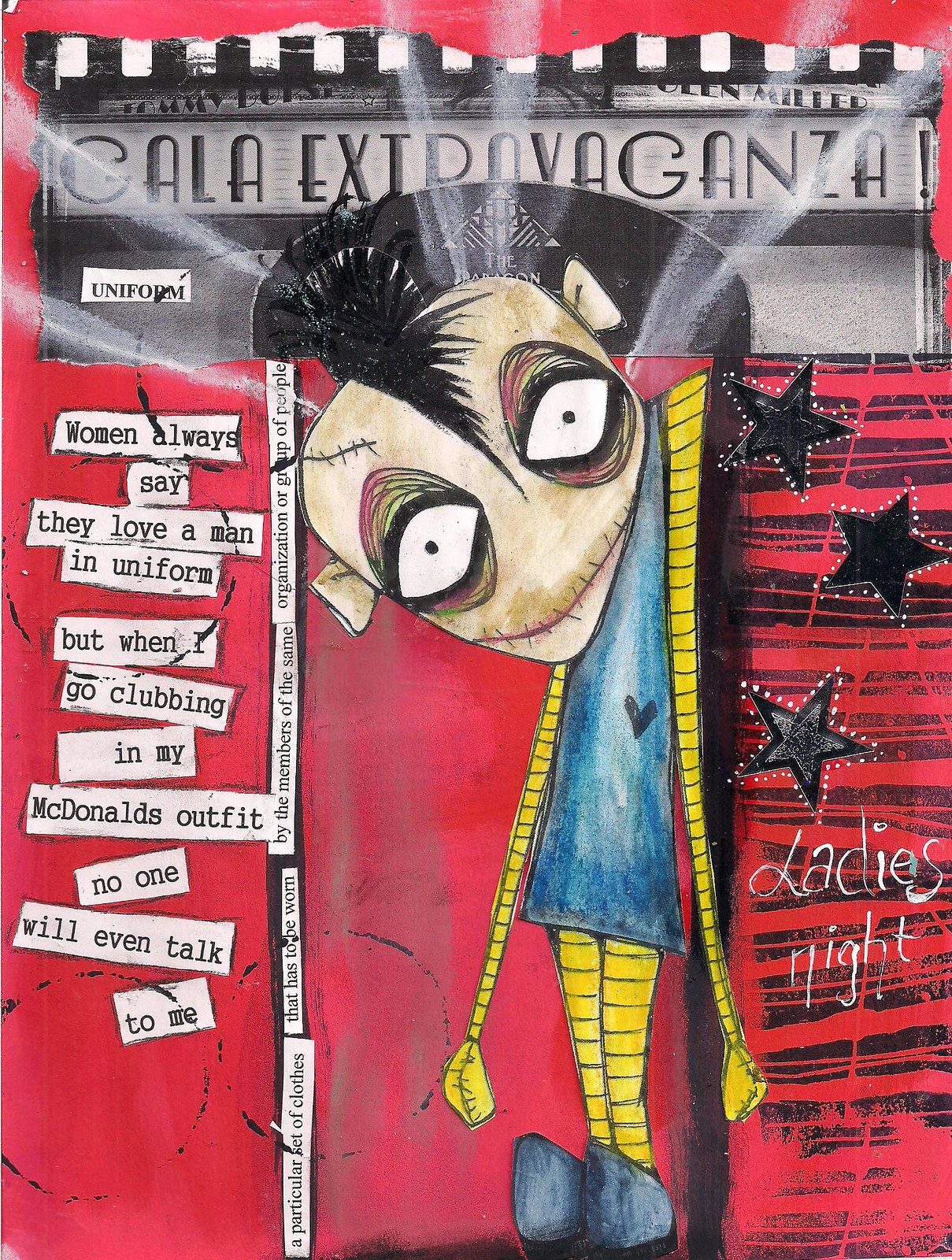In this image, there is a striking and eerie drawing of a doll with a narrow body, wearing a blue dress and long yellow striped sleeves and leggings. The doll features large eyes with rings around them, a stitched-shut mouth, and a black mohawk. The background is predominantly red with pieces of paper taped to it. At the very top, in bold black text, it says "Kala Extravaganza." To the left, there is a vertical series of typewritten text clippings that read, "Uniform, women always say they love a man in uniform, but when I go clubbing in my McDonald's outfit, no one will even talk to me." On the right side, there are three black stars and the words "Ladies Night" in white. The overall style resembles something you might see from the animated series "Invader Zim."